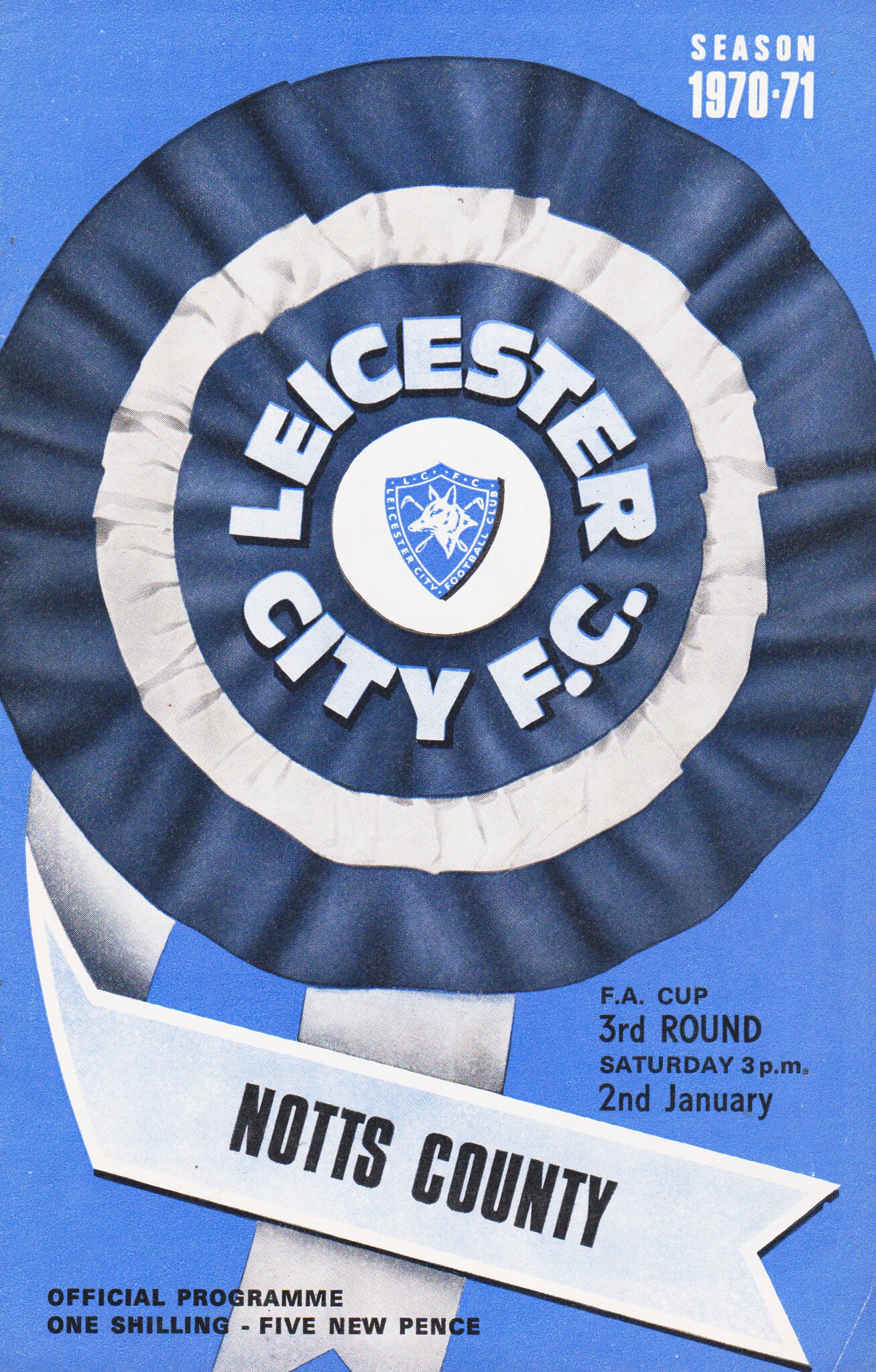The cover of this official sporting event program features a solid blue background dominated by a centrally positioned ribbon, resembling a prize ribbon, with alternating blue and white fabric. The ribbon's design includes a round fabric configuration that alternates blue and white edges, with a central white circle displaying a shield. The shield, shaped like a curved triangle with two additional sides at the bottom, contains the image of a wolf's head facing left with crossed golf clubs behind it. Encircling the shield within the white circle is the text "Leicester City FC" in white font. 

At the top right corner of the cover, "Season 1970-71" is printed in white text. Below the central ribbon, the text "F.A. Cup third round, Saturday 3 p.m., 2nd January" appears prominently. Additionally, there is a smaller white ribbon that crosses and folds over at the bottom, featuring the inscription "Knotts County." The bottom left corner of the cover contains the text "Official Program, one shilling, five new pence.”